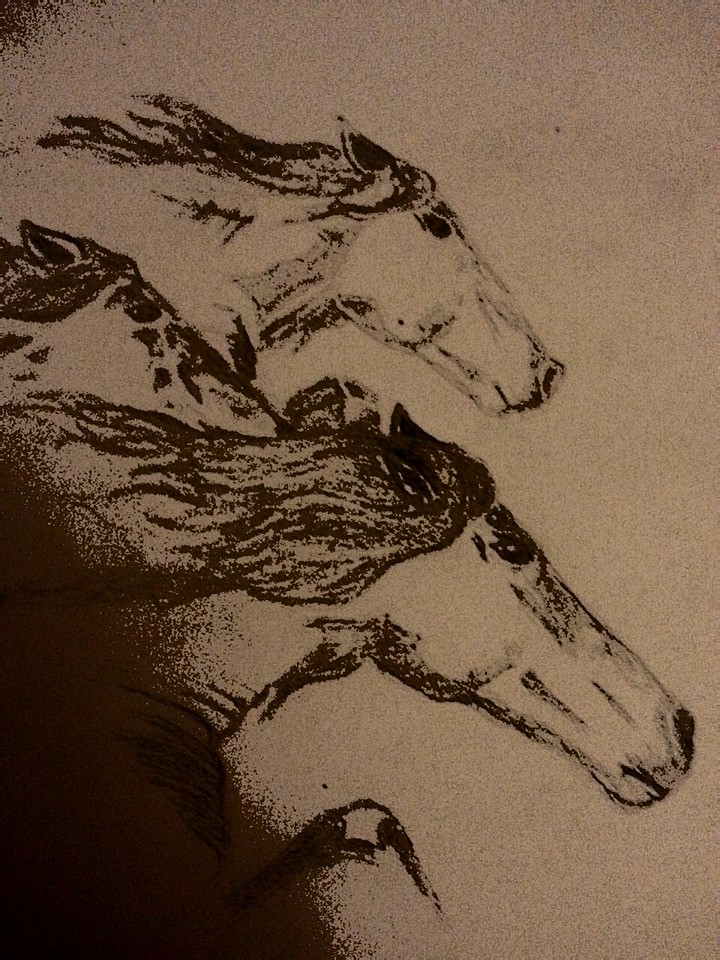The image features a detailed drawing of three horses set against a rough, pinkish-brown sketch pad or paper, which imparts a coarse and almost tan-reddish tone to the depiction. The horses are illustrated in mid-gallop and are viewed in profile, with their heads and manes prominently flowing as if caught in motion. All three horses are racing towards the right side of the frame, their bodies positioned such that their legs are not visible. This adds a sense of drama and movement to the image. The largest horse, closest to the viewer, leads the group, while the second horse follows slightly behind, and the third, shorter-nosed horse is positioned furthest back. The drawing is executed in dark-reddish ink, contributing to the richly detailed portrayal, which includes lines and dots adding texture to their manes. A shadow is present in the lower left corner, enhancing the depth, while there are no other obvious details, text, or markings to detract from the central scene of the racing horses.